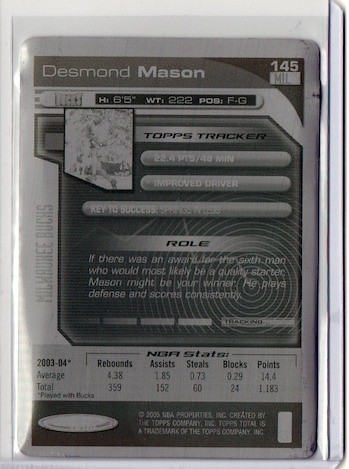This image is a detailed sports card in portrait mode with a predominantly white background and a silver border along the right. The card features black, gray, and white tones and showcases various statistics and information about the basketball player Desmond Mason. At the top, bold text reads "Desmond Mason 145 MIL." Below that, it lists his height as 6'5", weight as 222 lbs, and position labeled as FG, with additional text: "H65 WT222 POB F-G." 

The card includes a small, slightly blurry black-and-white illustration of Mason, which could potentially be a hologram. Further down, the card has a "TOPS tracker" section, indicating that Mason averages 22.4 points, with additional phrase stating "improved driver" and "key to success: springs and legs."

A narrative section suggests that if there were an award for the sixth man most likely to become a quality starter, Mason might be the winner, highlighting his consistent defense and scoring ability. The card specifies his affiliation with the Milwaukee Bucks during the 2003-2004 season and provides detailed statistics from that period: an average of 4.38 rebounds (total 359), 1.85 assists (total 152), 0.73 steals (total 60), 0.29 blocks (total 24), and 14.4 points (total 1,183). At the bottom, there's small print against a black bar, indicating "2005 NBA Properties Inc. Created by the TOPS Company, Inc. TOPS, TOTAL is a trademark of the TOPS Company, Inc." detailing that this card appears to be encased in a protective plastic sleeve.